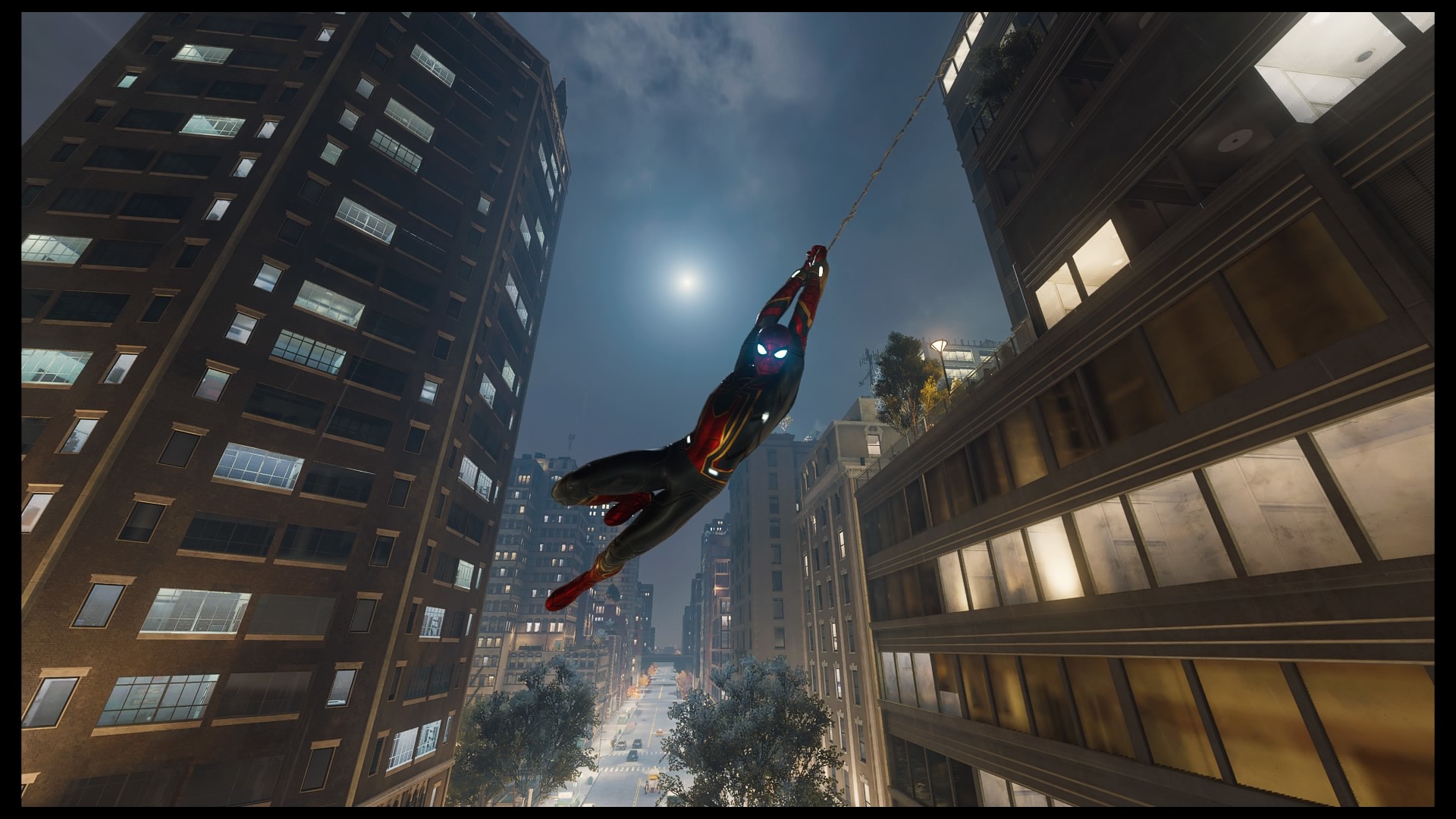This compelling image captures a scene that appears to be a screenshot from a Spider-Man movie. In the foreground, Spider-Man is dynamically swinging between towering high-rise buildings in what seems to be an urban environment. The building on the left, characterized by its unique hexagonal shape, features illuminated windows that add a sense of liveliness to the night scene. On the right, a more traditionally shaped square building also shows signs of life with lights glowing through its windows. 

Spider-Man, tall and lean, dons a striking costume in shades of red, gold, and black, accentuated by his signature red feet. His mask features glowing eyes, hinting at advanced tech or a heightened sense of alertness. Adding to the atmospheric quality of the image, the full moon glows behind Spider-Man's shoulder, casting a gentle light across the dark blue sky. Wisps of white clouds are scattered across the sky, completing the nocturnal vista and enhancing the dramatic tension of this urban escapade.